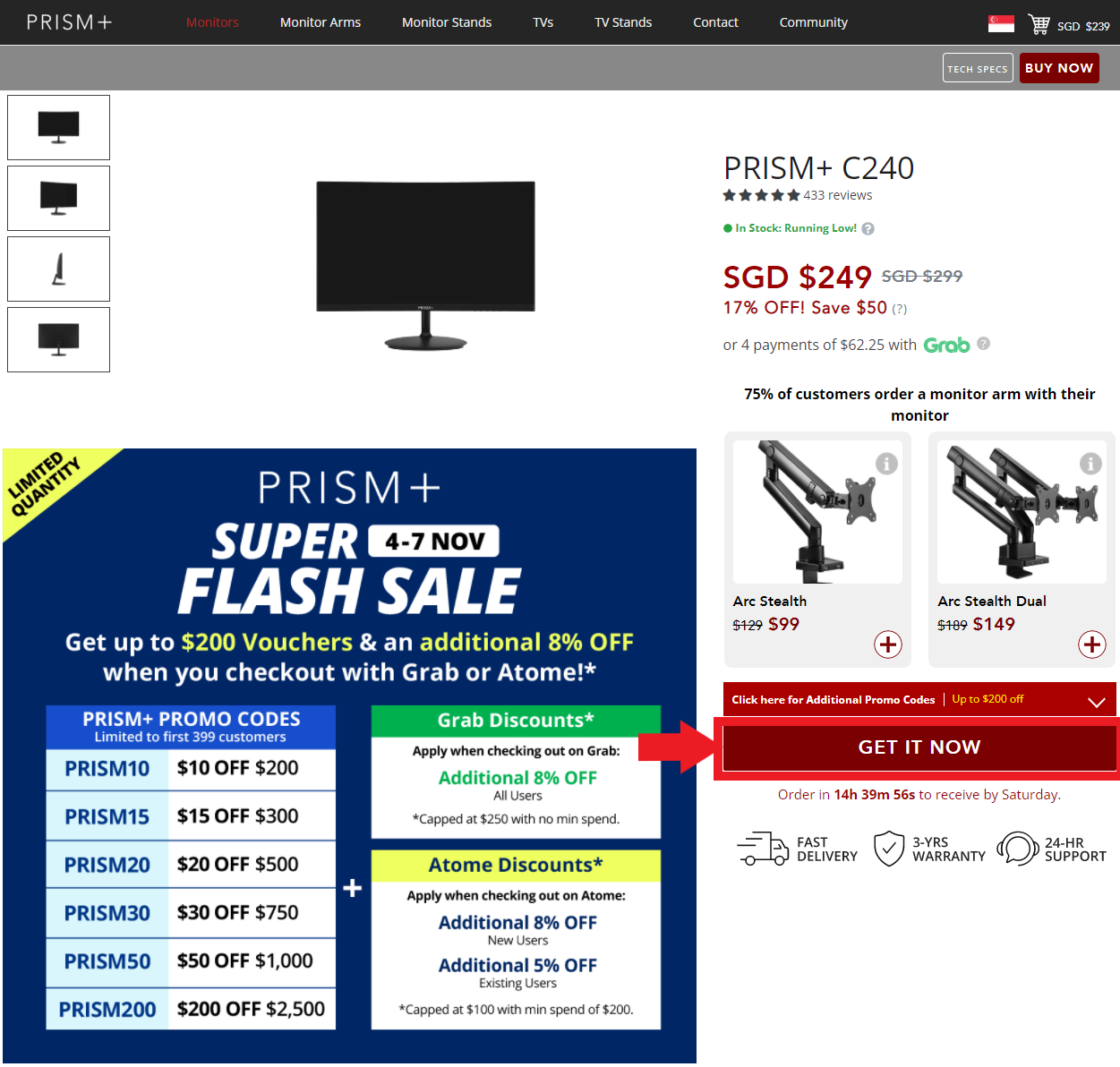This image shows a shopping page on the PRISM Plus website. The top of the page features a sleek black bar with white text serving as a menu. The menu options include PRISM Plus monitors, monitor arms, monitor stands, TVs, TV stands, contact, and community. In the upper right-hand corner, there is a shopping cart icon and a prominent red button labeled "Buy Now."

The center of the page showcases a product on a clean, white background—specifically, a computer monitor. Flanking the main image on the left are four smaller pictures of the monitor from different angles, providing a comprehensive view of the item. On the right side, the monitor's name and price are clearly displayed for potential buyers.

Below this section, there are images of two related products, each accompanied by their respective names and prices. Beneath these, a striking red button labeled "Get It Now" is highlighted with a red arrow and red outline, urging customers to take action.

In the lower-left corner, a banner ad announces the PRISM Plus Super Flash Sale, adding a sense of urgency and encouraging shoppers to explore potential discounts.